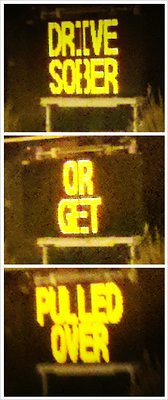A nighttime photograph captures a prominent road sign that sends a clear and urgent message: "DRIVE SOBER OR GET PULLED OVER." The sign itself is structured in a staggered format, with the phrase "DRIVE SOBER" displayed prominently, followed by "OR GET" on the next line, and "PULLED OVER" on the bottom line. The sign's background is black, creating a high contrast against the bright yellow, all-capital letter text. The bold, blocky font ensures that the message is easily readable, even from a distance. There is no cursive or decorative script, emphasizing the straightforward and serious nature of the warning. The photograph appears to have been taken at night, further highlighting the sign's importance for late-night drivers.